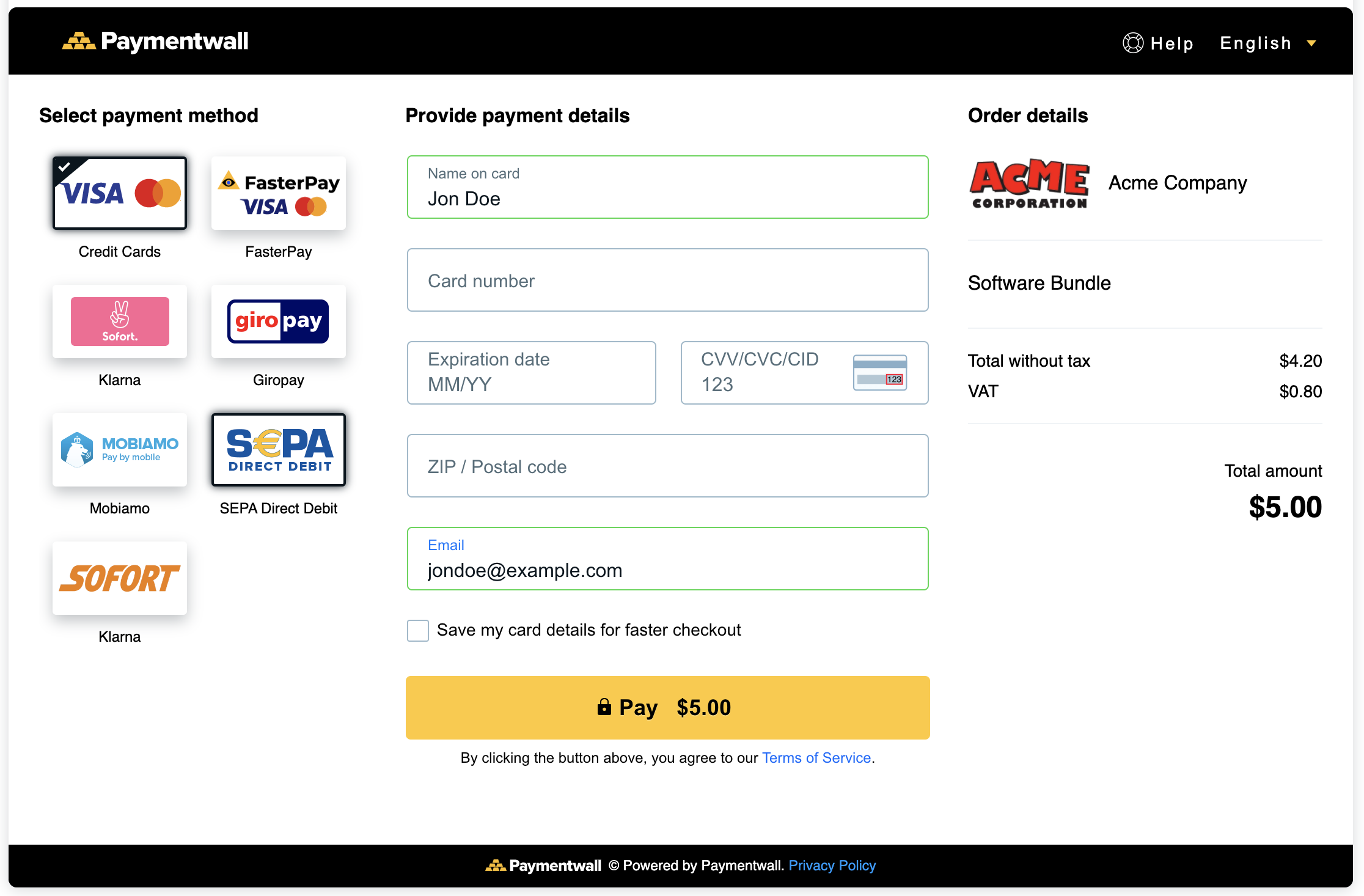This is a detailed screenshot of an online payment gateway interface. The webpage features a black band at the top and bottom, giving it a distinct framed appearance. 

On the left side, a small yellow triangle composed of dots is visible, possibly serving as a decorative element or indicator. The primary content in the center of the screen is primarily black text set against a white background.

At the top of the page, there is a navigation bar on the right-hand side that includes a help option and a language selection drop-down menu set to English. 

The left side contains a section for selecting a payment method with various payment options displayed in rectangular buttons. The options include Visa (currently selected), FasterPay, Mama, ShopPay, GyroPay, Mataz Modder, SEPA Direct, SOFORT, and Milano, though some of these names may be unfamiliar or misspelled.

In the center of the screen, there are fields to input payment details. These fields include:
- Name on Card: prefilled with "John Doe"
- Card Number
- Expiration Date
- CCV (security code on the back of the card)
- ZIP/Postal Code
- Email: prefilled with "johndoe@example.com"

Below these fields is an unticked checkbox labeled "Save my card details for faster checkout." 

At the bottom of this section, there is a prominent yellow button with black text that reads "Pay $5." Below this button is a note stating, "By clicking the button above, you agree to our terms of service."

On the right side of the screen, there's a summary of the purchase, including:
- The merchant's name, Acme Company
- The name of the product, a software bundle
- Subtotal: $420
- Tax: $0.90
- Total amount: $5

Finally, at the very bottom of the page, there are links to "Privacy Policy" and a disclaimer that the service is "Powered by Payment Wall."